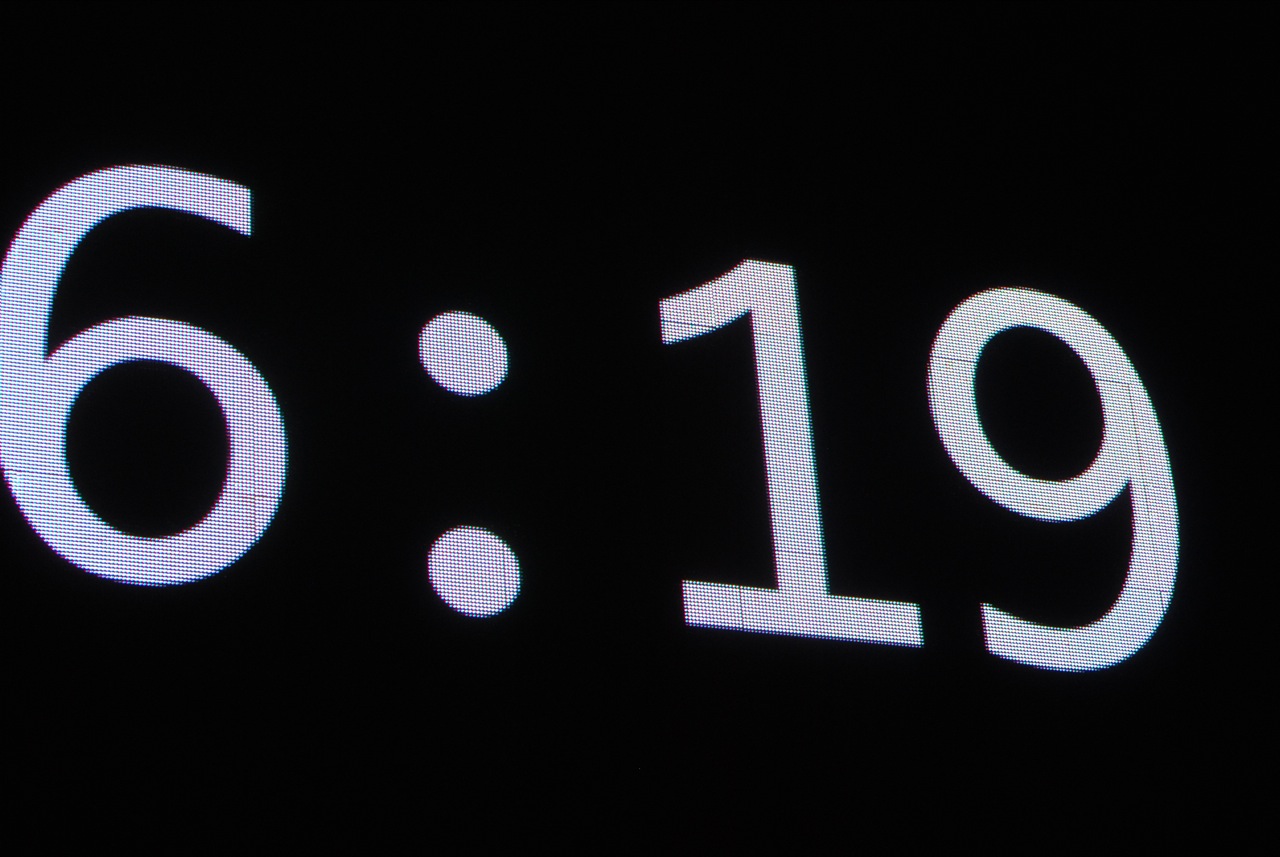The image captures a simple, close-up display of the time "6:19" on a solid black background. The numbers are large, white, and displayed in a digital, LED-like format. Each numeral is typical of those found on clocks or watches, and the display suggests it may be part of a larger screen, as slight vertical and horizontal lines are visible, indicating panel separations. The numbers, while straightforward in their design, are not perfectly aligned horizontally, with the "6" slightly higher than the "1" and "9," creating a gentle downward slope from left to right.